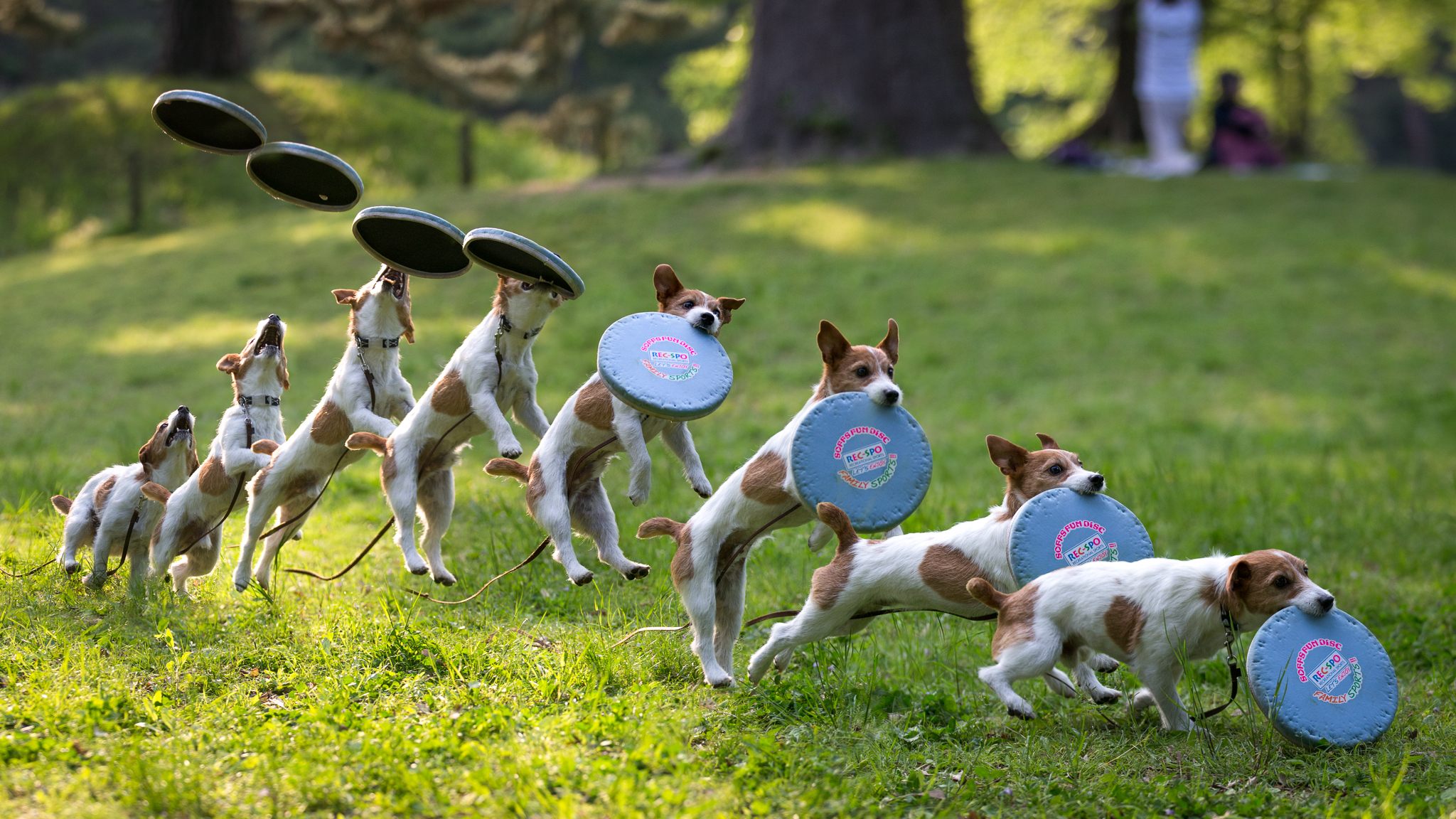In a vibrant park with sprawling green grass and gentle hills, a series of frame-by-frame images capture a lively scene of a brown and white spotted Jack Russell mix breed dog in action. The sequence begins with the dog on the ground, eyes locked on a blue frisbee soaring towards it. The next frames show the dog's agile leaps, propelling higher and higher, until it finally catches the frisbee mid-air. The background features a large tree trunk and blurred figures of people, including someone in a white shirt and pants standing, and another person in black attire seated and possibly engaged in an activity like yoga or aerobics. As the dog gracefully descends with the frisbee clamped in its mouth, the vibrant text "Shops Fundusk" and "Rexpo" becomes visible on the frisbee, indicating it's from a sports company. The final frames depict the energetic dog landing and dashing off, frisbee securely held in its mouth, ready for another round of play.